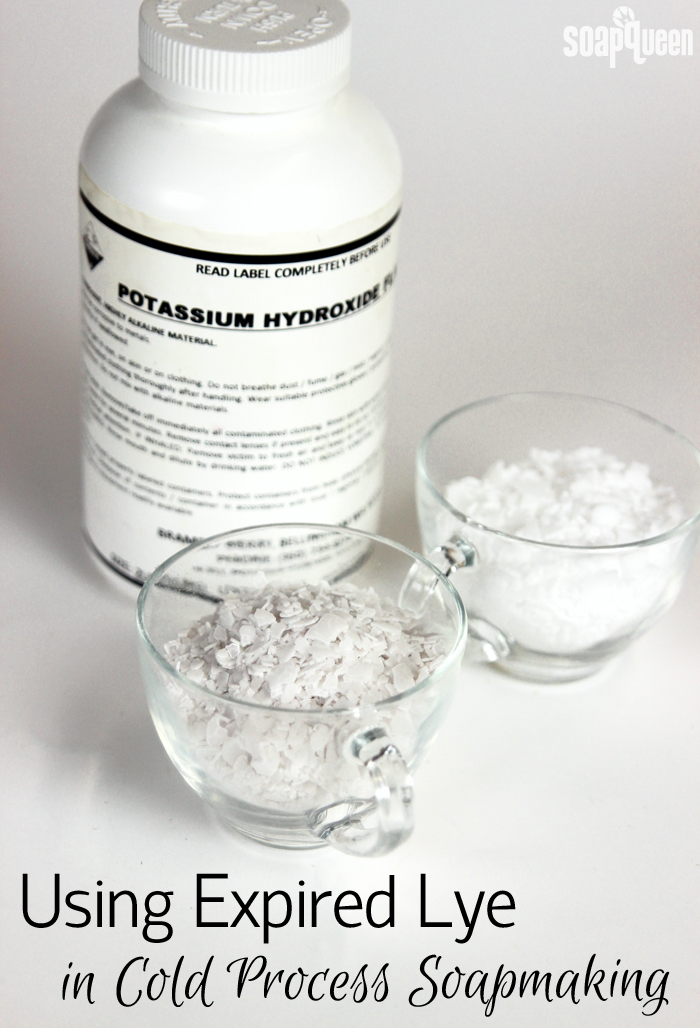This advertisement features a monochromatic photograph prominently displaying a white plastic bottle labeled "Potassium Hydroxide" in black text. Situated centrally, the bottle is accompanied by two small, clear mugs with single handles, placed to the left and right. Each mug contains distinct powdery substances: the left mug holds a gray powder, while the right mug contains a white powder, both having a flaky texture. Shadows cast by the mugs and the bottle are visible in the background, adding depth to the image. At the bottom of the page, the phrase "Using expired lye in cold process soap making" appears in black text, with "in cold process soap making" stylized in script. The top right corner of the advertisement is marked by the brand name "Soap Queen" in white lettering.